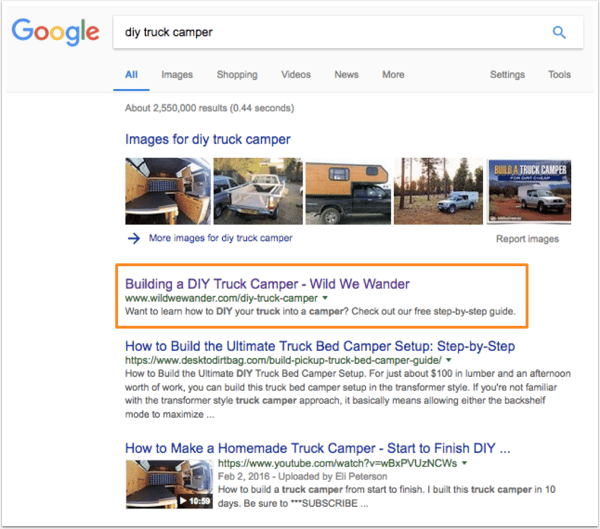Screenshot of a Google search page for "DIY truck camper." At the top, just to the right of the iconic multi-colored Google logo, the search query "DIY truck camper" is typed out. Below this, the navigation bar features options including "All," which is highlighted in blue, "Images," "Shopping," "Videos," "News," and "More." Toward the far right, there are options for "Settings" and "Tools." Just under the navigation bar, the search results begin, indicating the number of results found and the time taken to retrieve them. Below this, a section titled "Images for DIY truck camper" displays five thumbnail images of self-made truck campers installed in the beds of various trucks. Further down, there is a highlighted search result titled "Building a DIY Truck Camper - Wild We Wander," which invites users to learn how to transform their truck into a camper with a step-by-step guide. This search result is emphasized with an orange rectangle around the text, likely indicating the site the user was looking for.